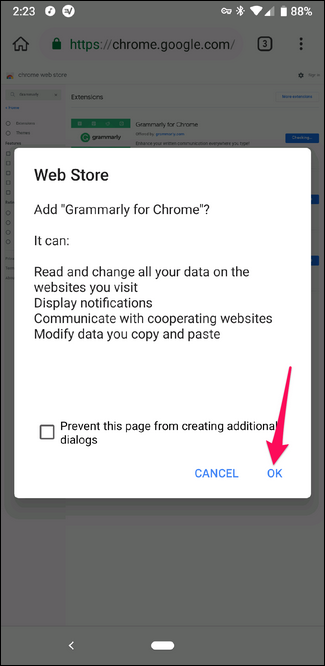The screenshot captures a webpage on a mobile device, identifiable by the status bar at the top displaying the time (2:23), battery percentage (88%), and icons for Bluetooth, mobile data, Wi-Fi, and battery status. The webpage itself, viewed in desktop mode on the Chrome browser, presents the URL https://chrome.google.com, indicating it's related to Chrome add-ons. The overlay on the page promotes adding the Grammarly extension to Chrome. The overlay details Grammarly's permissions, including reading and modifying data on visited websites, displaying notifications, communicating with cooperating websites, and altering copied and pasted data. A small checkbox option labeled "Prevent this page from creating additional dialogues" is present. At the bottom right, there are "Cancel" and "Okay" buttons, with a red arrow pointing to "Okay," suggesting user action is required to proceed with the Grammarly installation. The screenshot effectively demonstrates the process of adding the Grammarly extension to the desktop version of the Chrome browser.